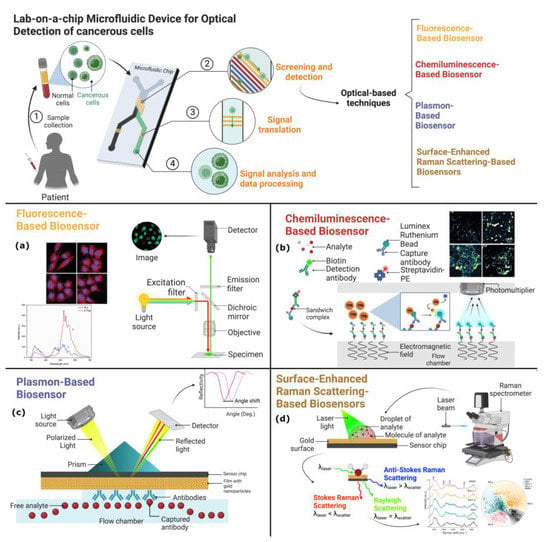The image is a detailed scientific diagram titled "Lab-on-a-Chip Microfluidic Device for Optical Detection of Cancerous Cells." It consists of several smaller panels arranged side by side and top to bottom, labeled from A to D. At the very top, there's an overarching title and a main illustration depicting a gray side profile of a man labeled "patient." This section also includes illustrations of sample collection from an injection into the hand, normal cells versus carcinoma cells, and a step-by-step breakdown from sample collection (1) through various processes.

Below this, panel A is titled "Fluorescence-Based Biosensor," featuring numerous graphs, numerical data, and diagrams such as excitation filters, light sources, detectors, emission filters, dichroic mirrors, objectives, and specimens. Panel B, labeled "Chemiluminescence-Based Biosensor," includes illustrations and detailed breakdowns of analyte reactions, biotin detection antibodies, sandwich complexes, and more, albeit the text is partially indecipherable. Panel C, "Plasmon-Based Biosensor," shows detailed diagrams of polarized light sources, prisms, reflected light, and detectors, among other elements. Finally, panel D, titled "Surface-Enhanced Raman Scattering-Based Biosensors," also contains intricate diagrams and graphs, though the specific details are harder to discern.

Throughout the image, there is extensive use of arrows, color-coded elements (black, white, gray, yellow, red, pink, purple, blue, and green), and annotations explaining each step and component of the microfluidic device and its applications in cancer detection.